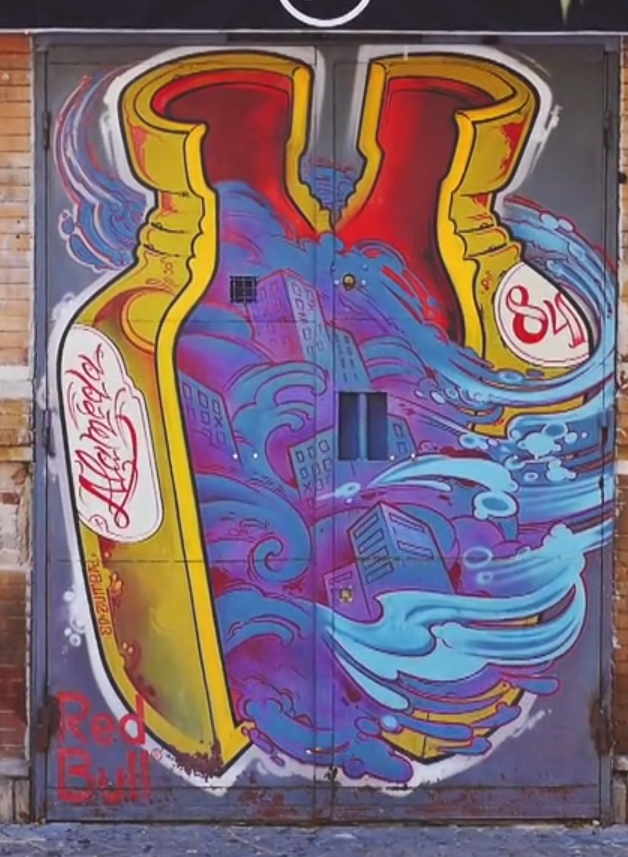The image depicts a graffiti mural on two large, dull gray metal doors set in a tan brick building, giving a vintage, industrial feel. The central focus of the mural is a gold bottle with a red interior, cracked open down the middle. Emerging from the split bottle are dynamic scenes of swirling ocean waves, clouds, and buildings, all rendered in shades of blue and purple. The bottle features red script logos on either side, one reading "Alameda" and the other with the number "84." In the bottom left corner of the doors, the words "Red Bull" are painted prominently. The mural showcases the artist's intricate design and vivid imagination, transforming the otherwise nondescript doors into a captivating visual story.